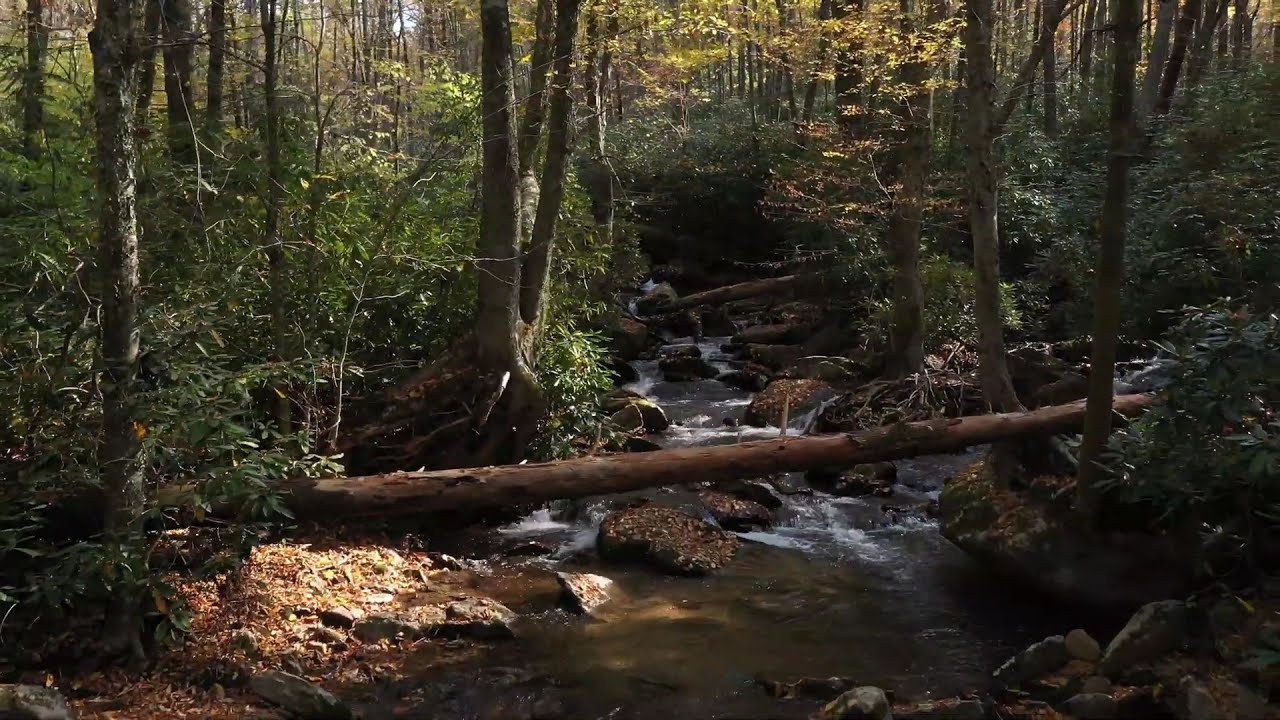This high-definition photograph captures a tranquil forest scene dominated by a stream, showcasing the serene beauty of nature. The stream, shallow yet flowing with purpose, winds its way from the mid-upper section to the bottom edge of the image, flanked by an abundance of rocks and several fallen tree trunks, creating natural bridges both in the foreground and farther back. The water, slightly murky with a hint of brown, cascades over the rocks, lending a touch of white from the froth. Lining the stream are tall, sturdy trees with a mix of green and yellow leaves, indicating the onset of autumn. Some trees stand proudly, while others have given in to time, laying across the stream. The scene is bathed in dappled sunlight filtering through the dense canopy, with sunbeams illuminating patches of the forest. The overall palette is rich with browns, greens, and yellows, and the forest, thick with shrubs and vegetative growth, extends into the background, creating a secluded, untouched nature setting. The absence of people emphasizes the pure, untouched essence of this picturesque woodland stream.